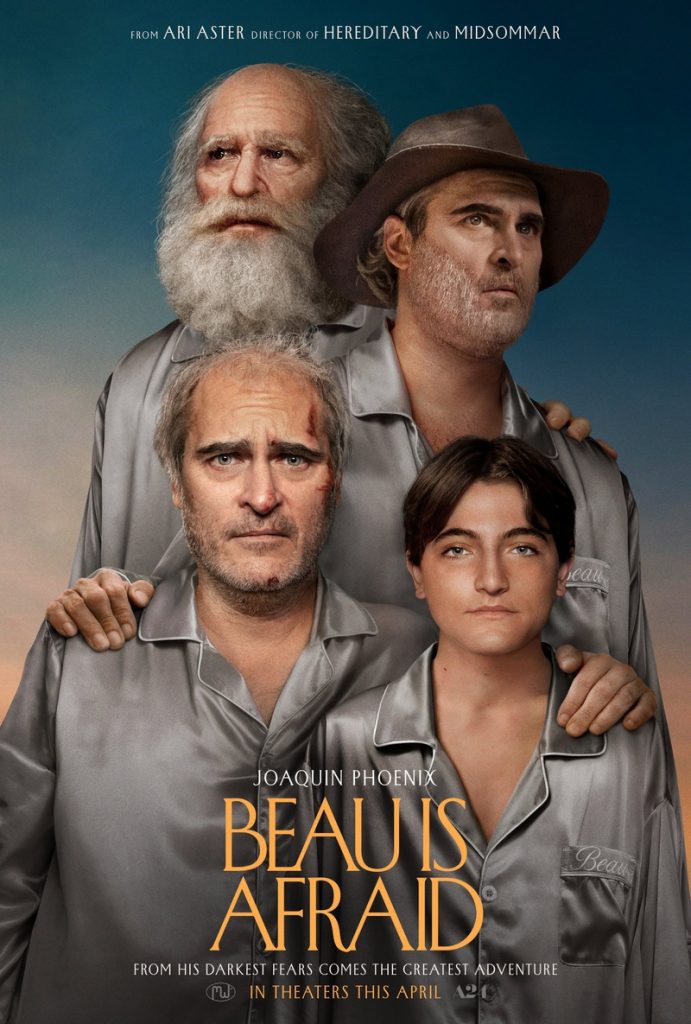The movie poster from Ari Aster, the acclaimed director of "Hereditary" and "Midsommar," showcases a haunting and intriguing scene. At the center, the bold yellow title "Bo is Afraid" stands out, with a white description below it reading, "From his darkest fears comes the greatest adventure in theaters this April." Four men are depicted, two at the top and two below, each pair seemingly reflecting older and younger versions of the same individuals, possibly indicating a journey through different stages of life. The top left figure is an older man, balding with sparse gray hair and a full beard reaching his chest. Next to him, on the right, is another older man with a hat reminiscent of Indiana Jones, sporting gray stubble on his chin. Below them, the two younger men look directly at the viewer. The man on the left is bald with short stubble, and on the right is the youngest figure with dark brown hair parted in the center. All characters are clad in satin gray pajamas, adding an eerie uniformity to the composition. Additionally, at the bottom of the poster, the name "Joaquin Phoenix" appears prominently in white, linking the renowned actor with this dark, adventurous tale.